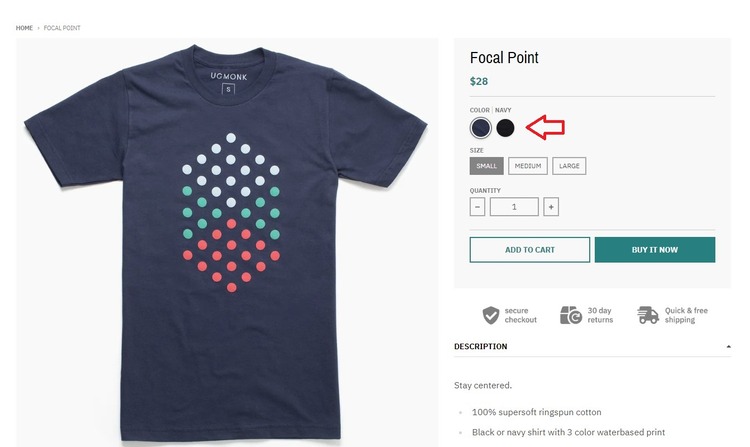Screenshot of an e-commerce purchase page showcasing a navy blue t-shirt with a geometric pattern of white, aqua, and pink polka dots arranged in a non-uniform diamond-like shape. The t-shirt takes up the left side of the screenshot against a white background. To the right, there is a product description, listing the brand "Focal Point" and pricing the shirt at $28. Customers can choose between two colors, navy or black, and select sizes ranging from small to large, with small currently selected. Below the size options, there is a "Buy It Now" button highlighted in teal and an "Add to Cart" button in white. Additional product details mention that the shirt is made from 100% super soft ring-spun cotton and features a three-color water-based print. This page is for purchasing the t-shirt, not for designing it.